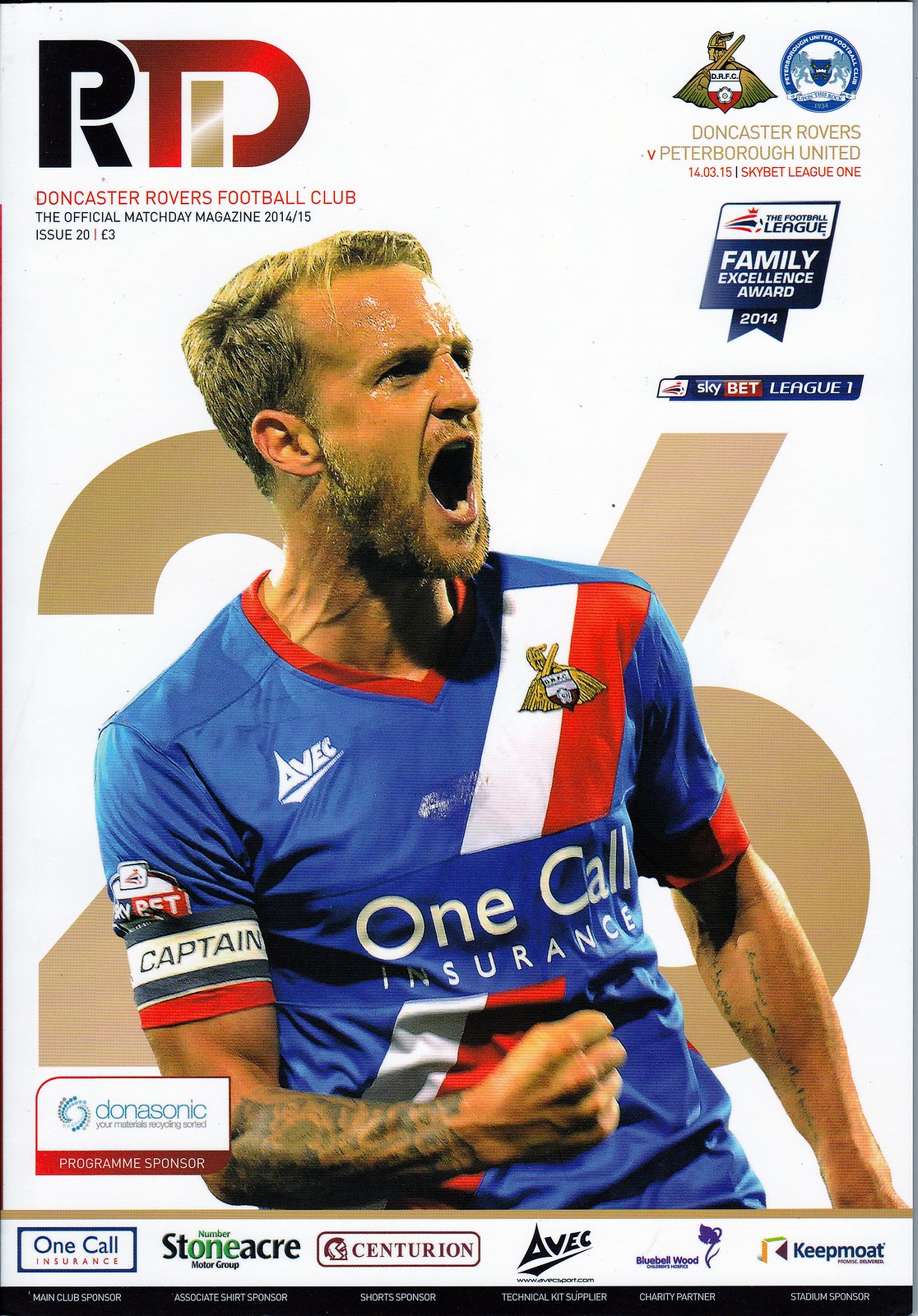This image depicts the cover of the official match day program for the Doncaster Rovers Football Club, issued for the 2014-2015 season. The background of the magazine is white with prominent elements aligned on both the left and right sides. On the upper left-hand corner, there is a large black “R” followed by a character that transitions from a “T” shape into a “D” shape, incorporating a gold eye between them. Below this, the text in red reads “Doncaster Rovers Football Club,” followed by “the official Match Day magazine 2014-15 issued 20” in black. Further below, in red, it says "Issue 20," and below that, in black, the price "£3."

On the upper right side, there's a gold Viking facing left, holding a white and red shield. Adjacent to this is a blue circular seal with white text that reads "Peterborough United Football Club upon the Rock 1934." Under this seal, in gold, are the words "Doncaster Rovers versus Peterborough United." Further down, in red, it displays "140315 Skybet League 1." Below the Viking, there is a logo for the Football League, accompanied by the text “Family Excellence Award 2014” and “Skybet League” at the bottom.

Dominating the center of the cover is a photograph of a Caucasian man, the team captain, depicted from the waist up. He is energetically yelling in celebration with his fist pumped across his chest. He has tattoos on his forearms, a beard, and short, golden blonde hair. He is wearing a blue jersey with red cuffs and collar, and the text "One Call Insurance" is emblazoned across the chest. The right arm of his jersey bears the captain’s designation. Behind him, in gold, the number “26” is visible. Along the bottom of the cover are advertisements for Donasonic, Stoneacre Motor Group, Centurion, AVEC, Bluebell Wood, and Keepmoat, tagged with “promises delivered” beneath.